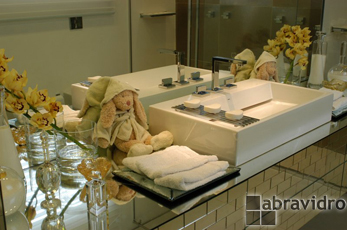The image features a carefully arranged bathroom scene. The background transitions from a greenish hue on the right to a slightly peach color on the left, eventually deepening into a darker green. On the right-hand side, there are dainty cups holding vibrant yellow flowers with orange centers encircled by thin black lines.

A plush stuffed animal, sporting a green hat, sits on a glass countertop, its light tan fur and reddish-tan nose subtly highlighting its label. In front of it, pristine white towels are neatly folded. To the left, a pristine white sink holds a strainer with white items, likely bars of soap, on the edge. The entire arrangement is beautifully reflected in a mirror positioned behind the sink.

On the right-hand side, another stuffed animal is placed alongside more of the yellow and orange flowers. The lower right-hand side of the scene includes a decorative tile pattern featuring brown, reddish, and greenish tiles. Three dark gray squares with white shadows surround the word "A-B-R-A-V-I-D-R-O" in matching gray and white-shadowed lettering, completing the detailed tableau.